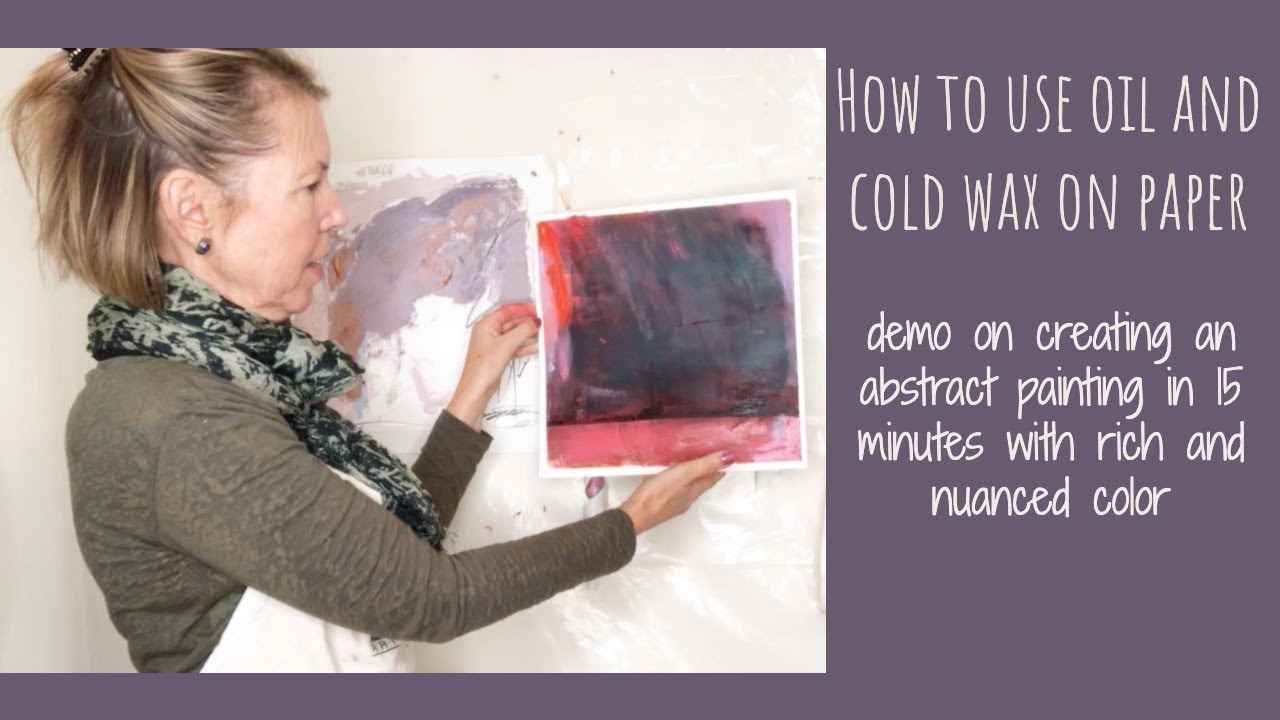In this detailed photograph, an older white woman with short blonde hair held up in a clip and styled in a bob stands against a white wall. She wears a dark green shirt, a white apron to protect her from paint, and a green and gray abstract-print scarf around her neck. She is holding up two pieces of abstract artwork on paper—a vibrant composition in red, black, and dark purple hues and a pastel piece featuring light purple and pink tones. To her right, a purple text box with white lettering reads, "How to Use Oil and Cold Wax on Paper: Demo on Creating an Abstract Painting in 15 Minutes with Rich and Nuanced Color." The background also includes a hanging painting with light purple and pink abstract art, complementing the instructional and creative ambiance of what appears to be a video tutorial thumbnail.